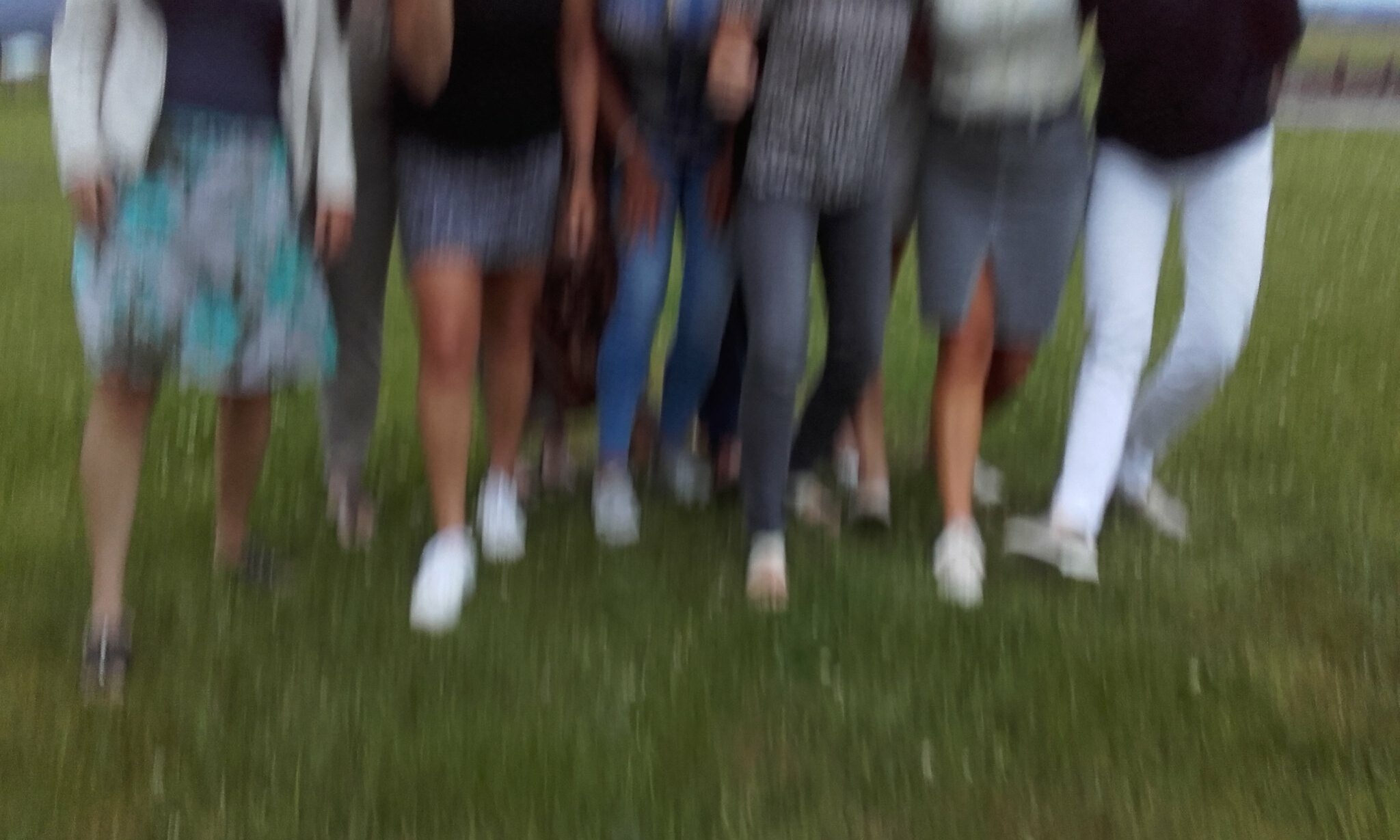In this blurry outdoor photo taken in a grassy field, about eight or nine people are captured from the shoulder down, mostly standing in a line with a couple standing slightly behind the rest. The attire of the individuals varies: one person is wearing a long-sleeved white sweater coupled with a teal dress adorned with a floral design, another is in a black shirt and gray shorts, followed by someone donning a blue shirt and blue jeans. The next individual is wearing a gray shirt and black jeans, while another is dressed in a tan shirt with a gray miniskirt. On the far right, there's a person in a black shirt and white jeans. The focus of the photo is on the lower halves of the people, showcasing their legs and feet, providing a casual glimpse into their diverse fashion choices.